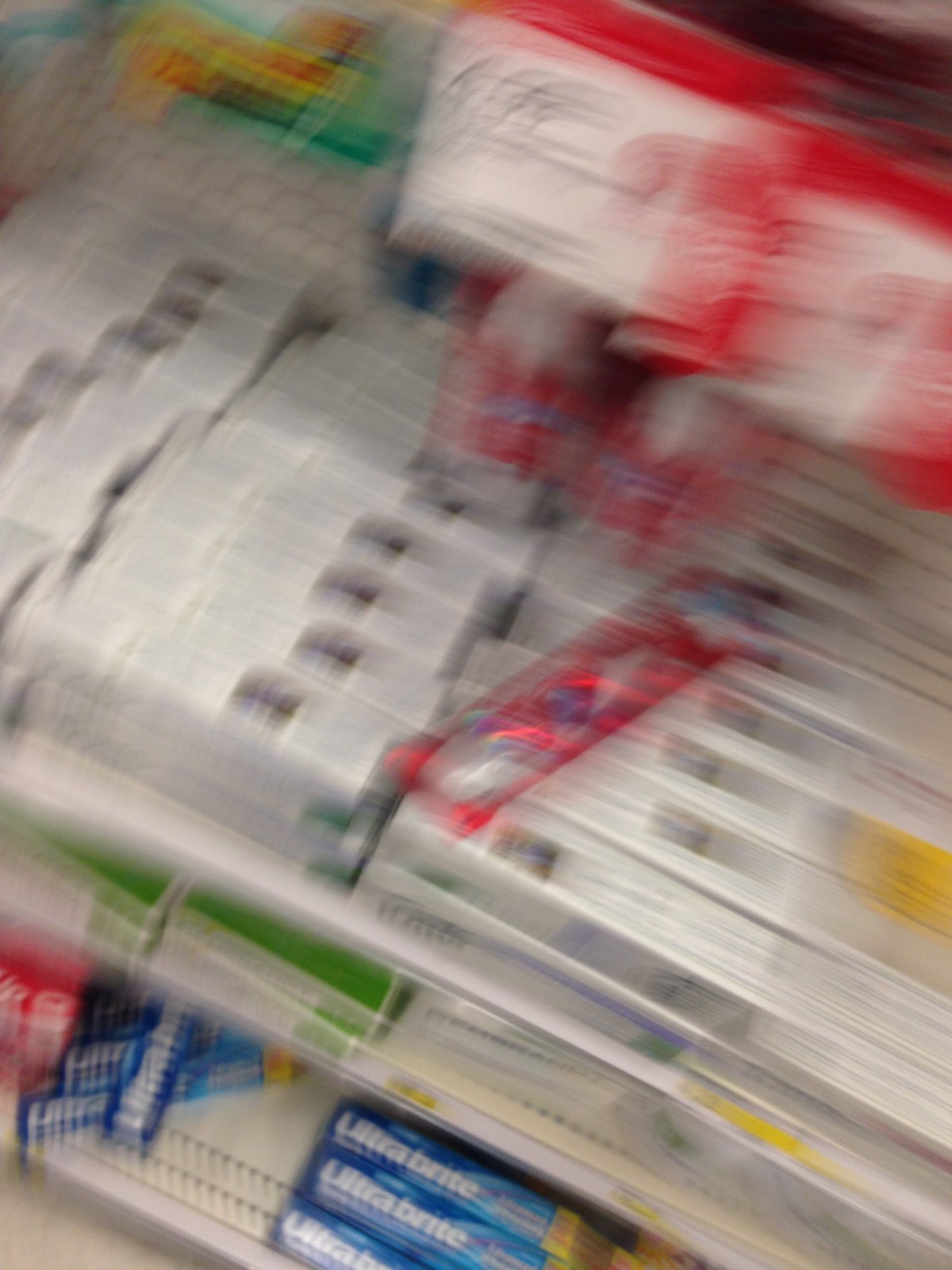The image appears to be taken in a grocery store or similar retail setting, although it is very blurry. The focus is on shelving units stacked with different kinds of toothpaste. On the top shelf, white boxes of toothpaste are stacked two or three high and several rows deep. Notably, there is a red object lying on top of these white boxes, possibly having fallen from an overhanging shelf above. 

The middle shelf features green boxes of toothpaste, while the bottom shelf displays red boxes on the left, which may be Colgate, and blue boxes labeled "Ultra Bright." The arrangement suggests a full display dedicated to dental care products. Despite the poor image quality, the details indicate a variety of toothpaste brands organized on three distinct shelves.